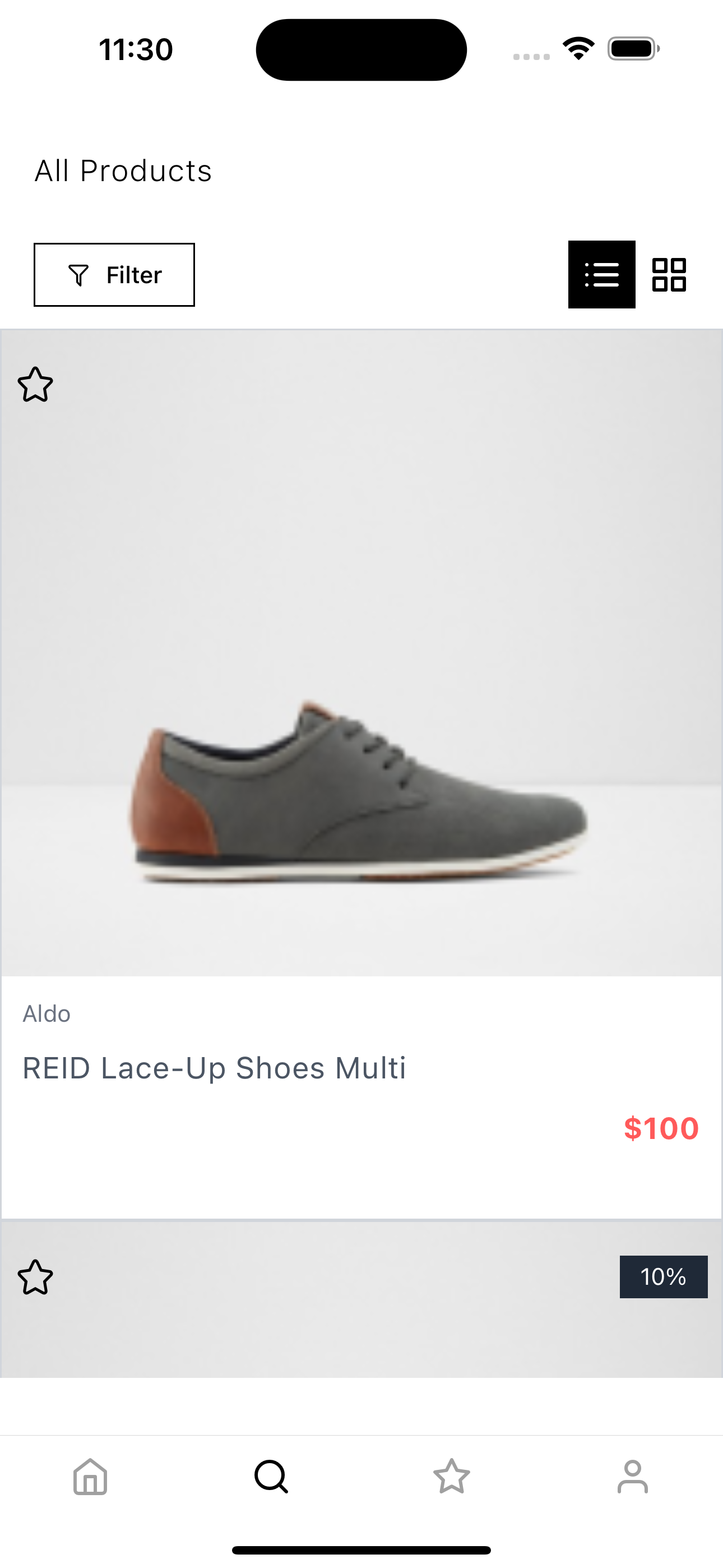Screenshot of a digital storefront showing a detailed view of Aldo Reed Lace-Up Shoes. The shoes are predominantly gray with a striking brown leather section at the back. The product is listed as "Aldo Reed Lace-Up Shoes Multi" and is priced at $100, displayed in red text. At the top-right corner, there is a row of three horizontal dots indicating additional options. Beneath the product title, a sleek black rectangle features a filter icon, allowing users to refine their searches. A gray bar contains a star icon labeled with "10%" in white, possibly suggesting a rating or discount. The bottom navigation bar includes icons for a home, search (represented by a black magnifying glass), favorites (a star), and user profile, with a solid black bar situated in the middle bottom section of the screen.